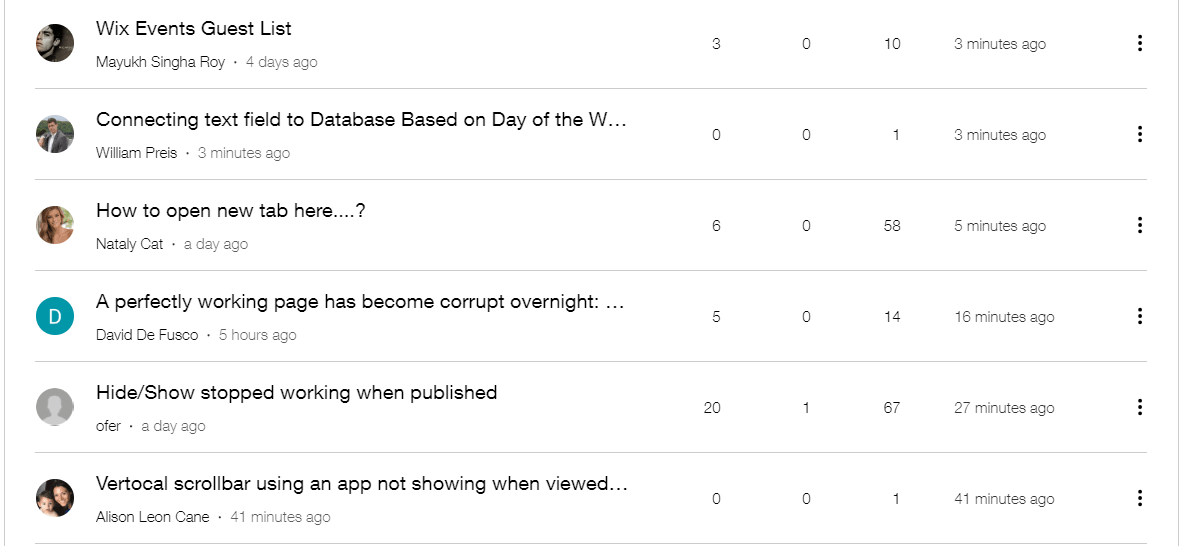This web page displays a list of six accessed results along with their associated details. Each result is identified by an icon on the left, which could be a picture of the person, an identifying letter, or a generic profile head and shoulders icon. 

1. **WIC’s Events Guest List**
   - **Author:** Mayuka Singa Roy
   - **Time:** 4 days ago
   - **Metrics:** 3, 0, 10
   - **Last Activity:** 3 minutes ago
   - **More Options:** Three vertical black dots on the right

2. **Connecting Text Field to Database Based on Day of the Week**
   - **Author:** William Priest
   - **Icon:** Mail photo
   - **Time:** 3 minutes ago
   - **Metrics:** 0, 0, 1
   - **Last Activity:** 3 minutes ago
   - **More Options:** Three vertical black dots on the right

3. **How to Open New Tab Here?**
   - **Author:** Natalie Cat
   - **Time:** 1 day ago
   - **Metrics:** 6, 0, 58
   - **Last Activity:** 5 minutes ago 
   - **More Options:** Three vertical black dots on the right

4. **A Perfectly Working Page has Become Corrupt Overnight**
   - **Author:** Dave DeFusco
   - **Time:** 5 hours ago
   - **Metrics:** 5, 0, 14
   - **Last Activity:** 16 minutes ago
   - **More Options:** Three vertical black dots on the right

5. **Hide/Show Stopped Working When Published**
   - **Author:** Ofer
   - **Time:** 1 day ago
   - **Metrics:** 21, 0, 67
   - **Last Activity:** 27 minutes ago
   - **More Options:** Three vertical black dots on the right

6. **Vertical Scroll Bar Using an App not Showing When Viewed**
   - **Author:** Allison Leon Cain
   - **Time:** 41 minutes ago
   - **Metrics:** 0, 0, 1
   - **Last Activity:** 41 minutes ago
   - **More Options:** Three vertical black dots on the right